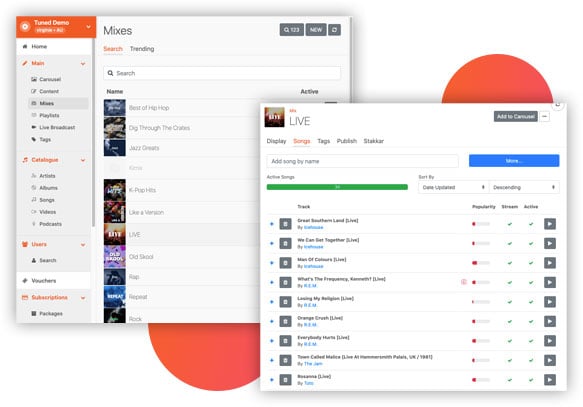Here is a refined and detailed caption for the dual-overlapping images:

---

The composition features two overlapping vertical rectangular images, each with a white background. The image on the right partially overlaps the image on the left, covering most of its left edge and top-left corner.

### Left Image:
The left image includes an orange rectangular header at the top, with white text reading "Demo." Down the left side, there is a vertical navigation menu:

- **Home** (in black)
- **Main** (in orange, accompanied by a pull-down menu)
- Several small, unreadable categories in black
- **Catalog** (in orange with a pull-down menu), followed by:
  - Artists (in black)
  - Albums (in black)
  - Songs (in black)
  - Videos (in black)
  - Unreadable category (in black)
- **Users** (in orange with a pull-down menu)
- **Search** (in black)
- **Vouchers** (in black)
- **Subscriptions** (in orange with a pull-down menu), followed by:
  - Packages (in black)

The main content of the first image includes a section titled "Mixes" (in black) at the top, followed by:

- **Search** (in orange)
- **Trending** (in orange)

Below these headings is a search box and subsequent listings with titles like "Best of Hip Hop" (in light gray), "Dig Through the…" (partial title), and "Jazz…" (partial title), next to small, indistinct images in the left column.

### Right Image:
The overlap image begins with the word **LIVE** in all caps at the upper left, adjacent to an album cover icon. Directly below are tabs labeled:

- **Display** (in black)
- **Songs** (in orange)
- **Tags** (in black)
- **Publish** (in black)
- An unreadable label in black

A horizontal rectangular box below these tabs invites the user to "Add song by name." To the right of this box is a bright blue button labeled **Menu** in white text.

Below these elements are sections:

- **Artist Songs** (with a "Sort By" option to the right)
- Two sort options ("Date Updated" and "Descending") 

Finally, the image includes a list of entries, each marked by turquoise or blue dots and featuring a vertical gray rectangle with a white "B" inside it. Adjacent to these markers are various details, presumably related to the songs or other media entries displayed.

---

This detailed caption captures the key visual and textual elements in both images, providing a comprehensive description for someone who cannot see the images.